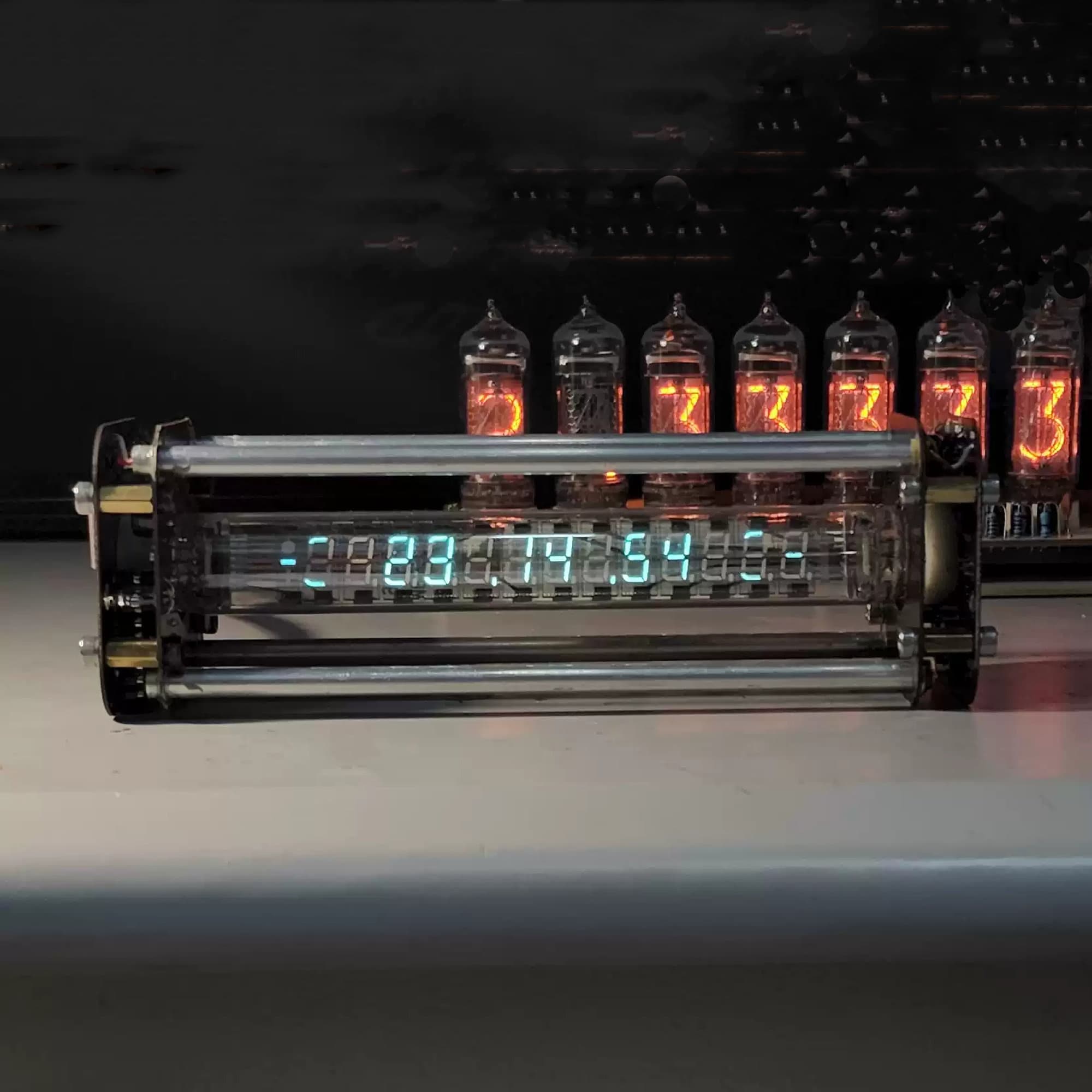The image depicts a distinctive setup of two clocks with markedly unusual styles, prominently positioned in the center of a square frame. The main clock occupies the central portion, taking up about half of the image. It features a digital, scientific calculator-like display with a numbers sequence "23.14.54," potentially representing a time in a 24-hour format. Above and below these digits are minus signs, reinforcing the clock’s scientific or technical appearance. Positioned behind this main clock are seven vintage Nixie tubes, each glowing with the number three, arranged closely together in a line, albeit one tube is not lit. 

The backdrop from the upper left to upper right corner is a black wall speckled with numerous light blue marks. Below this wall, there is a gray surface that stretches from the bottom left to the bottom right of the image. Resting on this surface, the main clock device is displayed on what seems to be a slate table. The overall composition and elements, including the mix of digital and Nixie tube technology, evoke a scientific or retro-tech ambiance, reminiscent of devices seen in vintage sci-fi themes like those in Steins Gate.